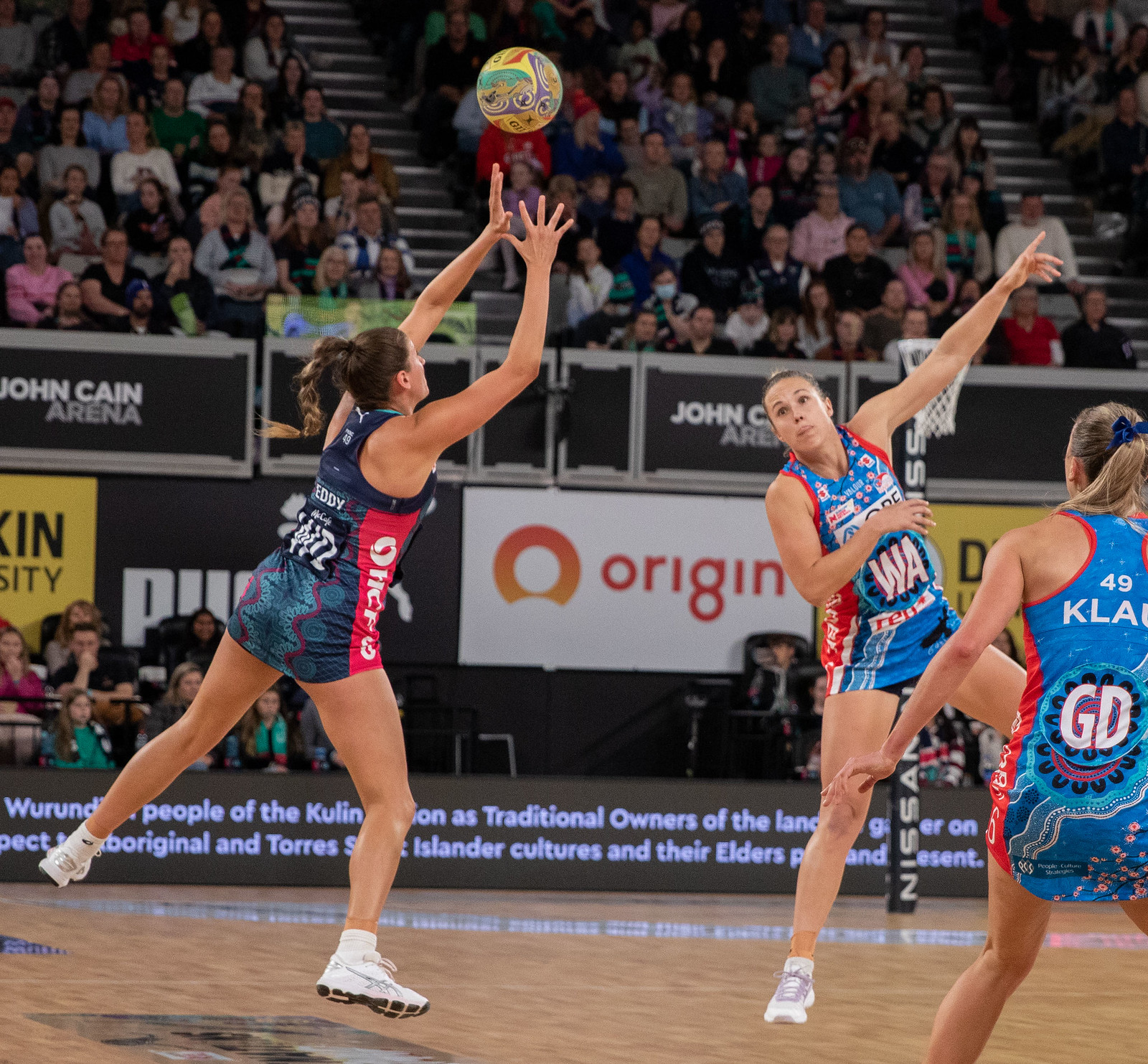The image captures a dynamic moment in a women's college indoor volleyball game held at John Cain Arena. The focus is on three players tussling for control of a colorful, swirled volleyball adorned with yellow, green, and purple patterns. The player on the left, identified by her dark blue and multicolored striped jersey and brown ponytail, is airborne with her arms extended, poised to either grab or hit the ball. Just to her right are two opponents in light blue and red outfits; one has her arm extended and a finger pointing up, while the other, identifiable by the number 49 on her back, has her hair tied back in a ponytail. The backdrop reveals a fully occupied stand of fans, mostly Caucasian, with several advertisements including Puma and Origin. The wall separating the crowd from the court is black with a gray border. The venue's name, John Cain Arena, is prominently displayed. The action unfolds on a typical shiny, brown gym floor.